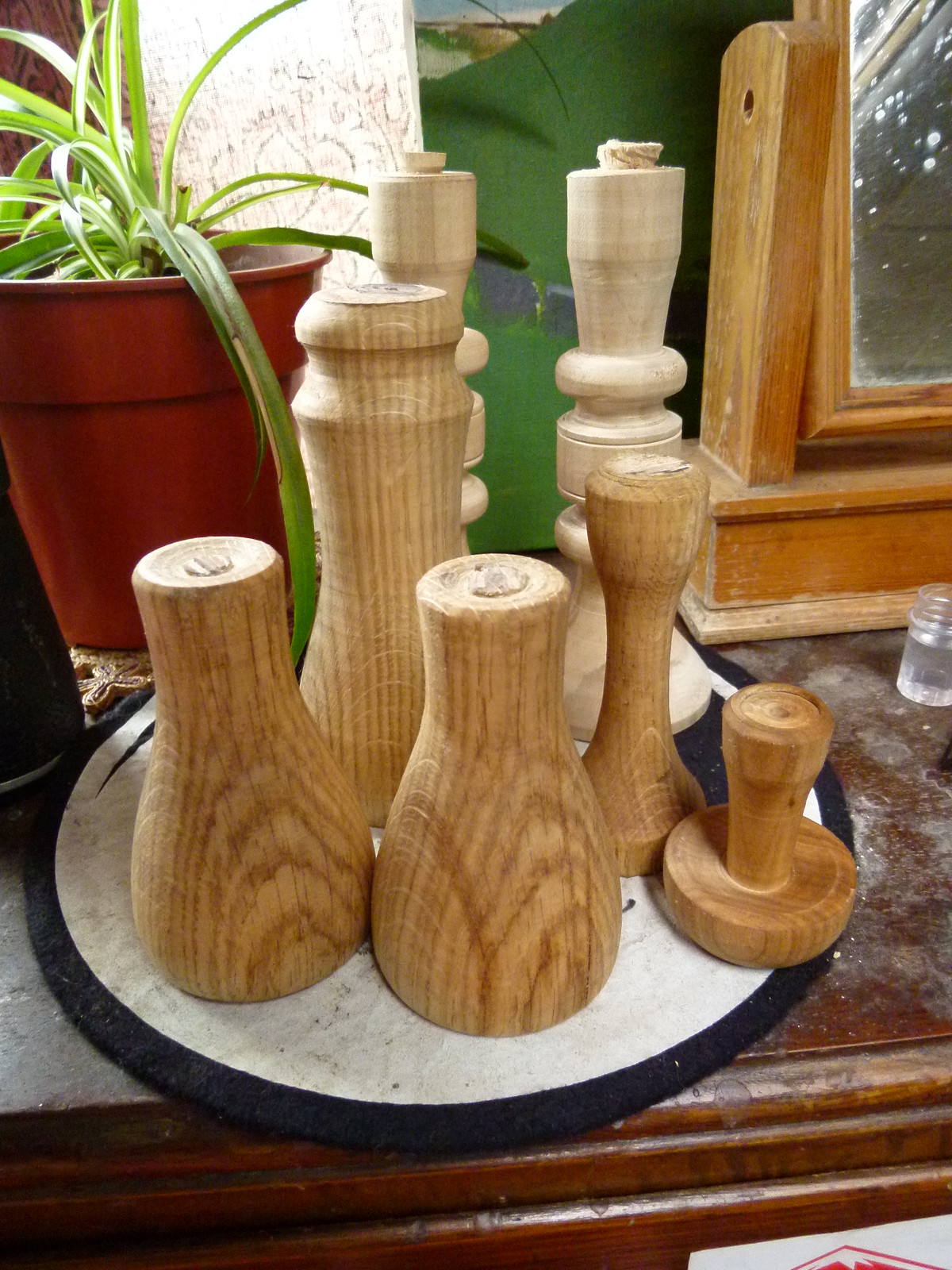The color photograph showcases a collection of wooden objects, possibly salt and pepper shakers or candlesticks, resting on a white tray with a black rim. The objects are lathe-turned and vary in height and wood finish, with the two tallest in the back made from light birch wood and the remaining five crafted from slightly darker wood. These handcrafted items, featuring cork or wooden plugs at the top, hint at an artisan's touch. The arrangement sits atop a round mat with a dark brown wooden surface possibly belonging to an antique vanity table, which may also have a leather top or cloth and talcum powder in view. To the far left, a terracotta pot with a lush green spider plant adds a pop of natural color, while in the upper right corner, a wooden-framed mirror with a pivoting arm is partially visible, capturing reflections from the vignette.